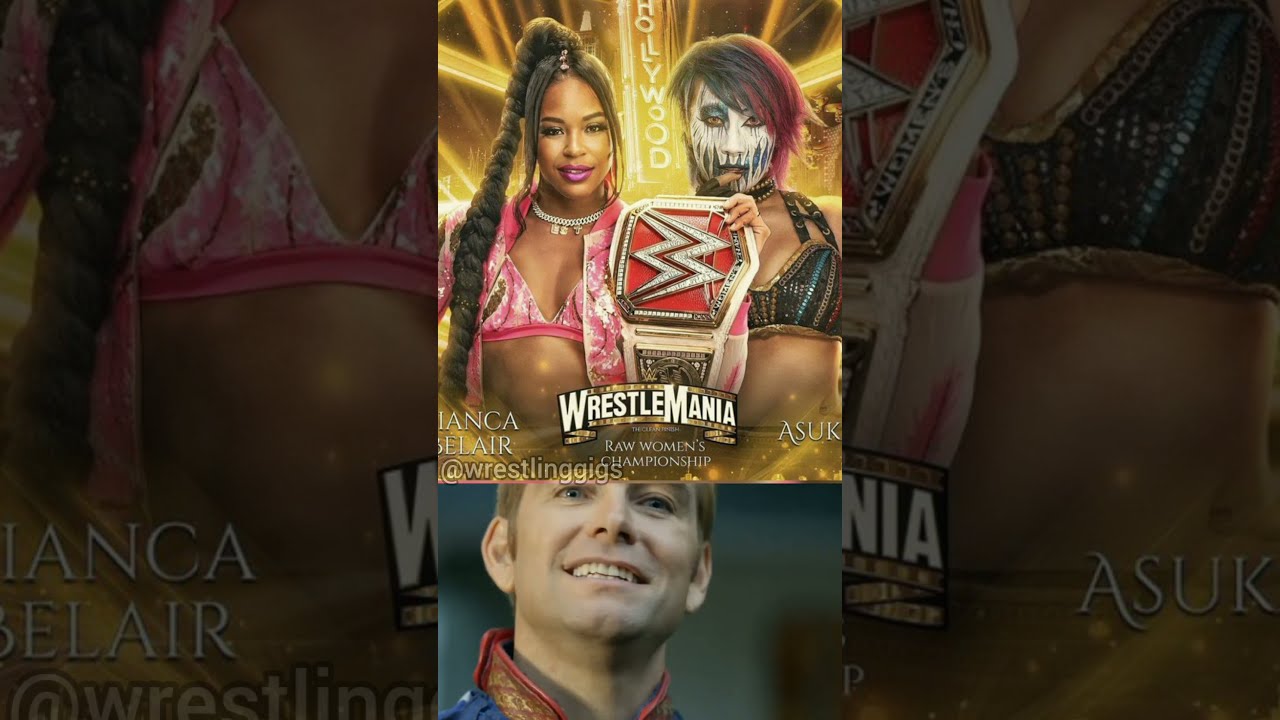The image appears to be a promotional poster for WrestleMania, potentially captured from TikTok or another social media platform. At the forefront, two WWE wrestlers are prominently featured, posing confidently in front of the iconic Hollywood sign. To the left stands an African American woman with a glossy pink bikini-like wrestling top, complemented by a matching pink jacket and silver chain. Her long, intricately braided ponytail cascades down her side, and her vibrant pink lips add to her striking look.

To her right is a woman with short red hair brushed to one side, her face covered in intricate white makeup with blue vertical stripes, giving it a skeletal appearance. She's donned in a black, studded bra adorned with various colored stripes—blue, gold, and red—with gold trim elaborating the outfit.

Both women are holding a WWE championship belt between them, which is predominantly red with gold trimming and a diamond-studded WWE logo. The scene is set against a backdrop that features the words "WrestleMania" in bold white letters, with additional, less discernible lettering at the bottom, blending into the dark, shadowy background. The background also mimics the appearance of a wrestling ring illuminated by neon lights.

At the bottom part of the poster, there's a clip from the TV show The Boys, showing the character Homelander staring upward, presumably reinforcing the admiration or perfection of the wrestlers above him. This clever juxtaposition creates a humorous, fan-made meme that seems to praise and celebrate the grandeur of the displayed WrestleMania image.